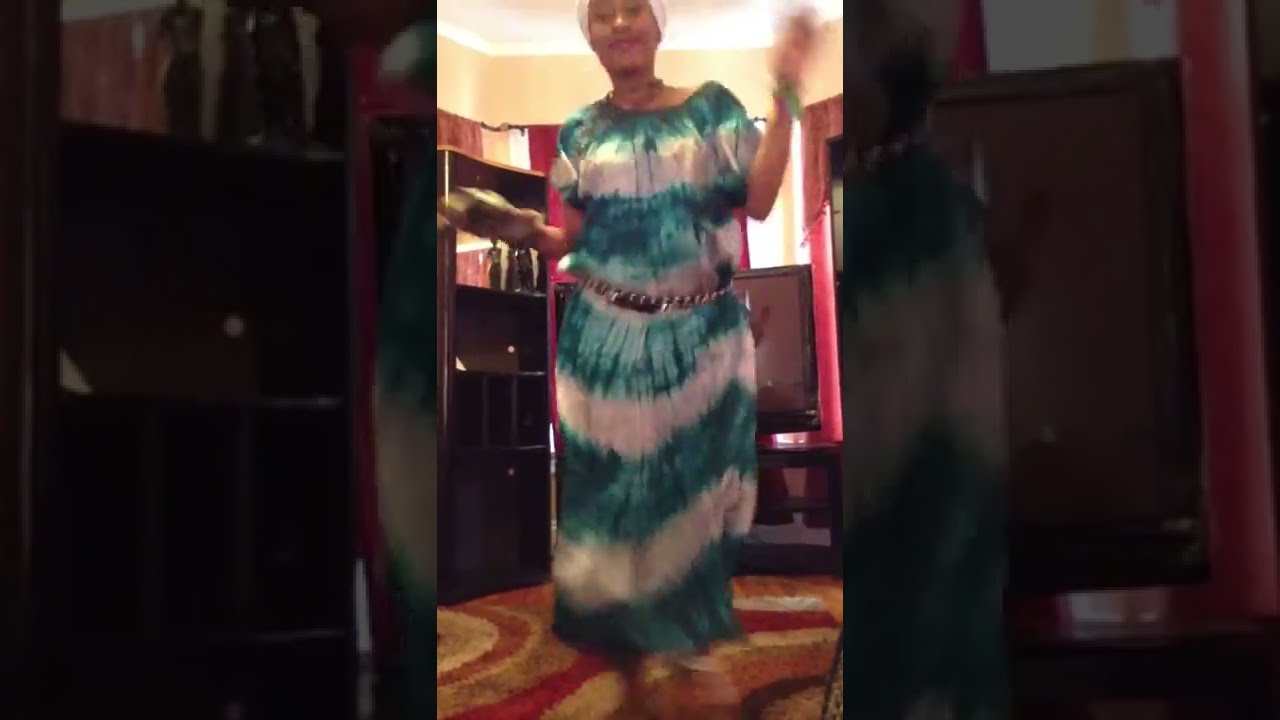A woman with brown skin, possibly African American, African, or South Asian, stands in the middle of a living room dancing on an orange and red swirl-patterned carpet. She is wearing a teal and white tie-dye dress with a fairly ornate dark brown or black belt adorned with silver metallic accents. Her head is covered by a white turban, and she is smiling while tossing her hips to the left. Both of her hands are raised, creating a motion blur. The room behind her is well-lit with daylight streaming through red-curtained windows on a beige wall. A 50-inch flat-screen TV on a short stand is directly behind her, partially obscured. To the left of the TV is a wood mahogany bookshelf, but the items on it are indistinct. The photograph is taken in portrait mode and is superimposed on a darker, broader version of the same image, emphasizing the central action of the woman dancing.